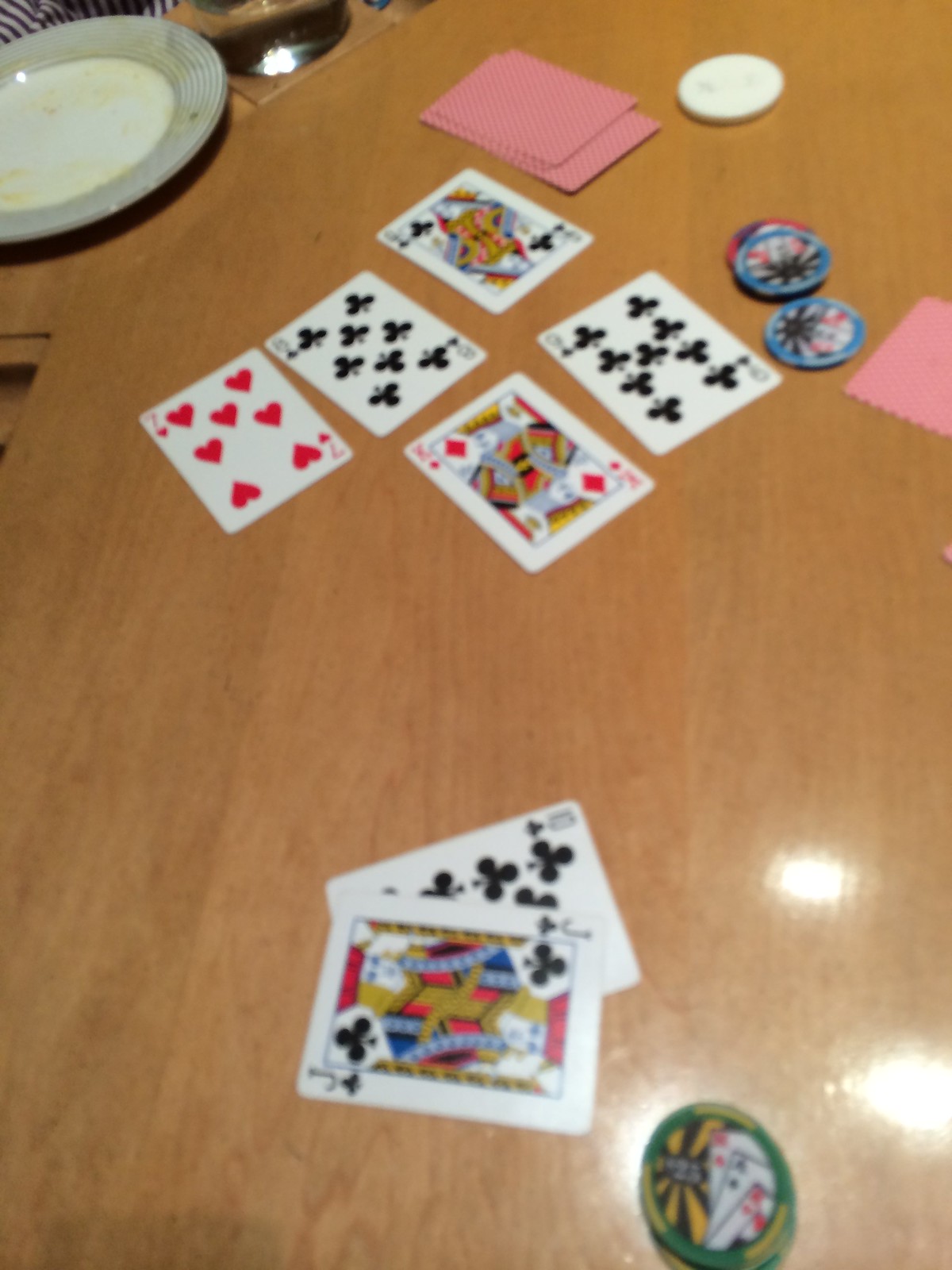In this image, starting from the upper left corner, there is a plate with a gray rim and a white interior. The plate has remnants of dried yellow food or possibly a dried yellow liquid. Below the plate, and to the left, there is a sequence of playing cards laid out: a white card with red hearts and the number seven, followed by a white card with black clubs and the number six, and next to them, a queen card. Just below this row is a king card with red diamonds and a nine of clubs card. Adjacent to these cards are two blue poker chips. Above the blue poker chips is a pink notepad, and to the right, there's a solitary white poker chip. Directly below the blue poker chips is another pink notepad. Moving farther down about three inches, there are two additional cards: a jack card is placed on top of a white card featuring the 10 of clubs in black text. Finally, at the bottom area of the image, there is a green poker chip adorned with black, yellow, and an image of three playing cards.